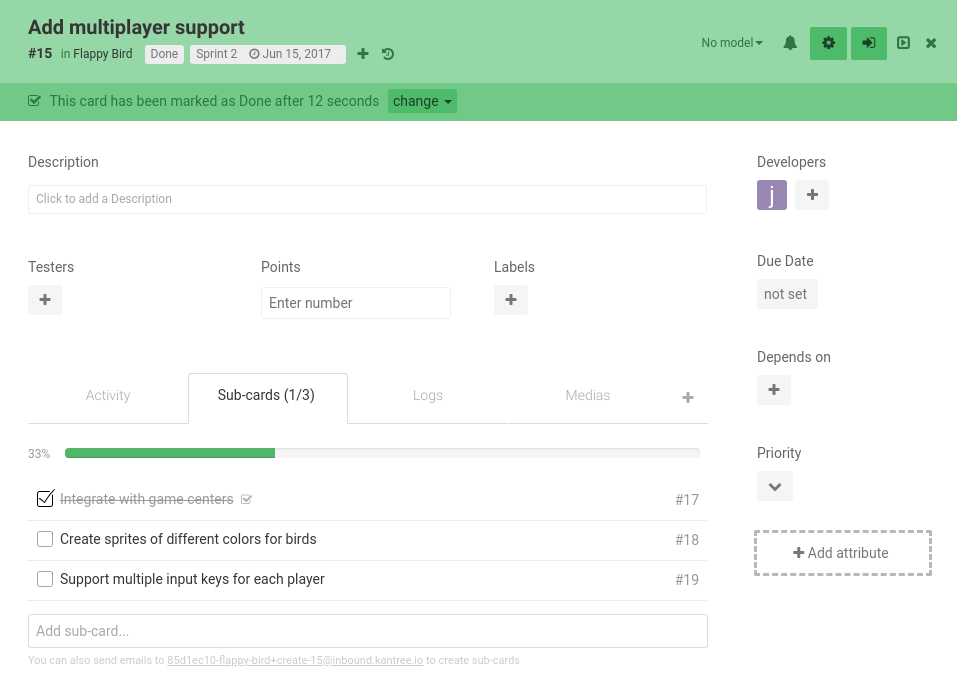The image showcases a user interface, possibly from a project management or task management application. In the center of the page, there is a task card with the title “Add multiplayer support,” ranked as number 15 and pertaining to the game "Flappy Bird". 

Below the title, there is a checkbox that has been ticked, accompanied by a note to its right that states: "This card has been marked as done after 12 seconds." 

At the top right corner, the interface includes several functional icons: a drop-down menu labeled "no model", a notification bell, a settings button, and an exit button.

Moving down the page, there are various input fields and buttons:
- A text field labeled “Description” with placeholder text “Click to add a description.”
- A section labeled "Points" with a text field below it prompting “Enter number.”
- An area for labeling developers with the abbreviation “G”.
- An adjacent “Add” button for including additional developers.
- A “Due date” field indicating that it has not been set.
- A dependency section labeled “Depends on” with an associated “Add” button.
- A “Priority” section featuring a drop-down menu.
- An “Add attribute” section with another “Add” button.

Each element and input field is designed to facilitate detailed project tracking and task management.